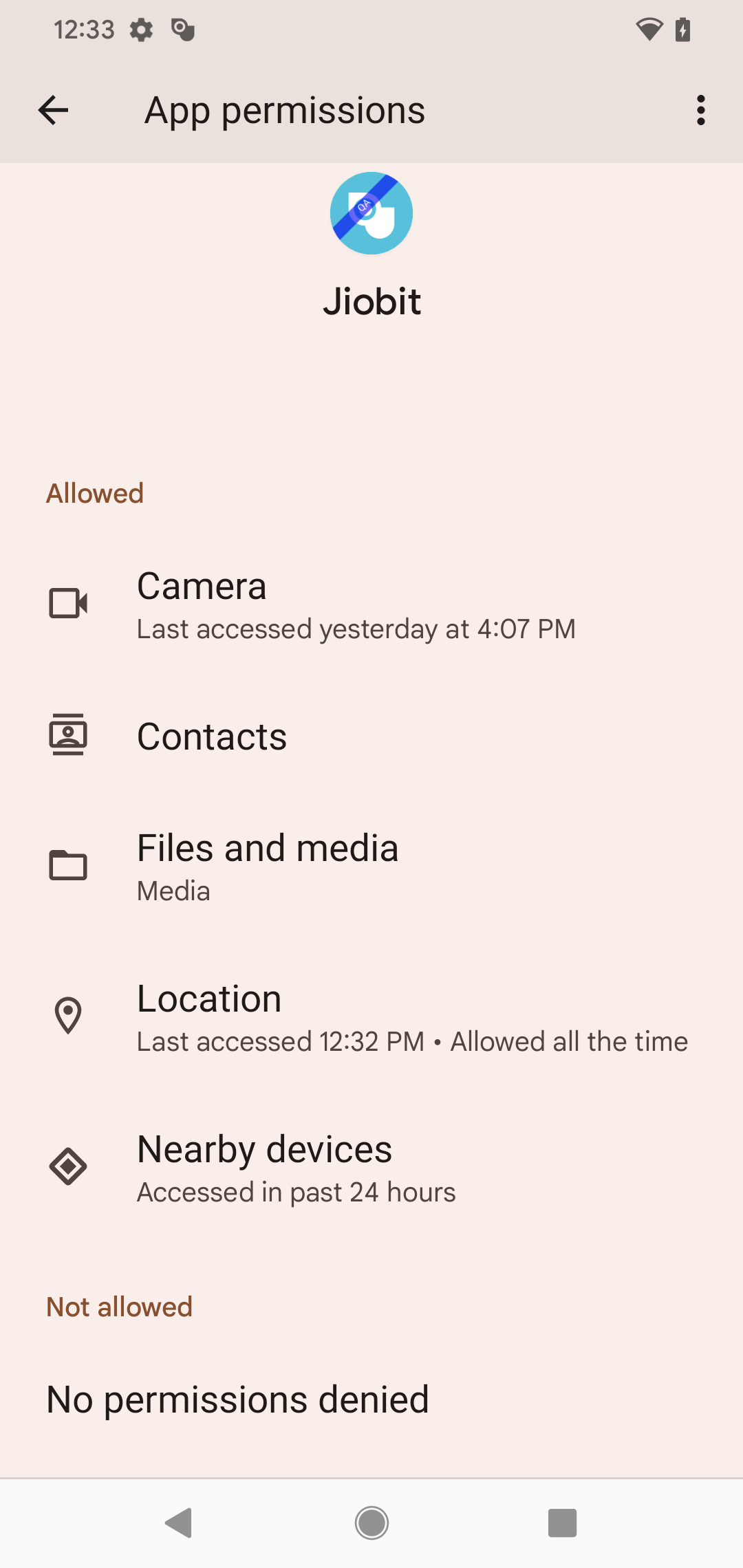The image depicts a detailed screenshot of a smartphone's permissions settings menu. At the very top, against a green backdrop, the notification bar displays the time "12:33," a gray cogwheel (settings) icon, and what appears to be a small gray rocket icon. Adjacent to these are the Wi-Fi and battery indicators.

Below the notification bar, there is a section encased in a tan and brown box. This section contains the title "Permissions," a back arrow, and a three-dot menu options icon.

The background of the main menu is tan, indicating that this is a sub-menu within the phone's settings. The screen provides detailed permissions information for an app named "JioBit," denoted by a teal and white circle with a blue line, and the name is written in black text.

Further down, there is a section labeled "Allowed" in brown text. Here, a list of permissions with corresponding icons and last accessed timestamps is displayed: 
- "Camera" with a camera icon, showing it was last accessed yesterday at 4:07 PM.
- "Contacts" with an icon resembling a TV screen and a cartoon person.
- "Files and media" with a manila folder icon.
- "Location" with a location pin icon, stating it was last accessed at 12:32 PM and is allowed all the time.
- "Nearby devices" with a square icon featuring a gray center, noting access within the past 24 hours.

Following this, there is another section labeled "Not allowed" in brown text, stating in black text, "No permissions denied."

At the bottom of the image, additional navigation icons are visible, including a back arrow shaped like a triangle, a gray circle, and a gray square.